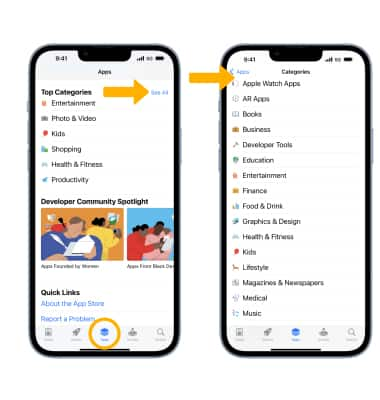The image features a clean white background with two smartphones positioned on either side. Both phones have a sleek black border and display a light gray section at the top, where various icons are visible. 

The smartphone on the left showcases a white area below the gray section. It prominently displays the text "Top Categories" followed by a list: "Entertainment," "Photo and Video," "Kids," "Shopping," "Health and Fitness," and "Productivity." A large orange arrow points to a blue hyperlink below this list. Beneath the arrow, the text "Developer Community Spotlight" is displayed alongside two small, blurry illustrations that seem to depict people and a family. Further down, the text "Quick Links" is shown with two additional blue hyperlinks beneath it.

The smartphone on the right also contains a similar layout. In the top left corner, a blue hyperlink is accentuated by another orange arrow pointing towards it. To the right of this arrow, a list including "Category," "Apple Watch Apps," "All Apps," "Book," "Business," "Developer Tools," "Education," "Entertainment," "Finance," "Food and Drink," and "Graphics and Design" is presented.